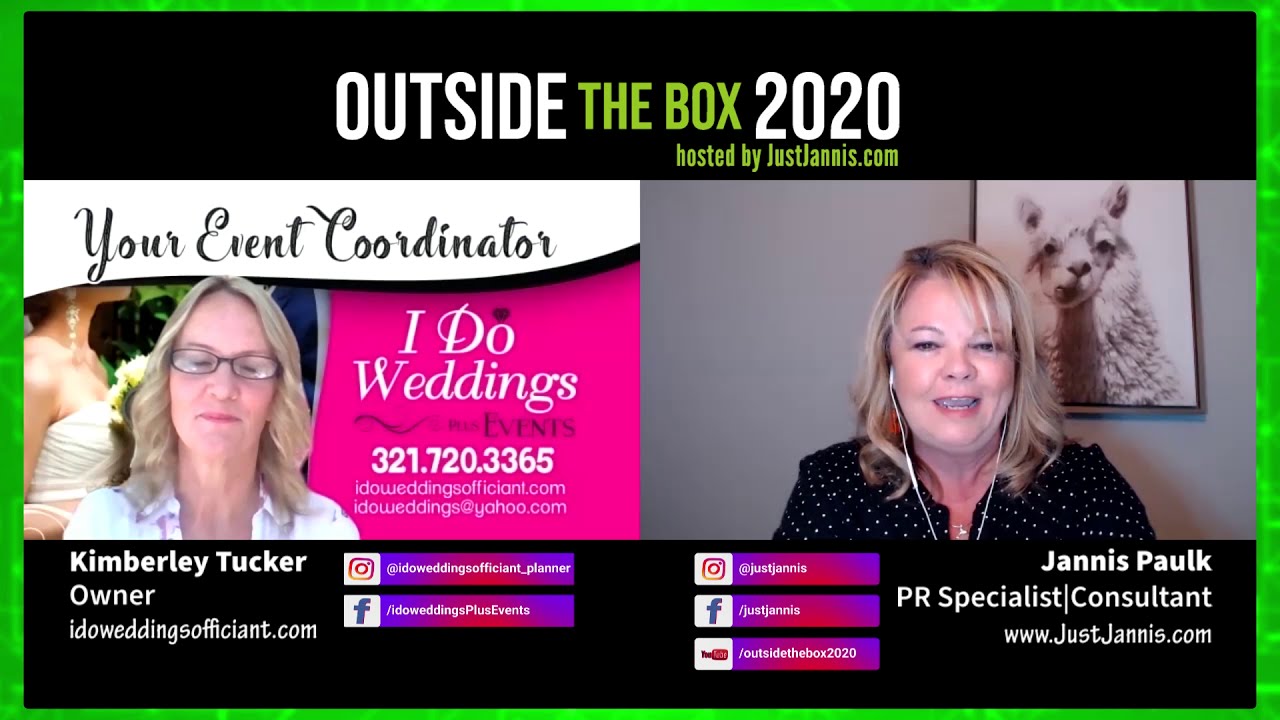The image is a promotional poster for an internet talk show called "Outside the Box 2020" hosted by justjanice.com. The vibrant design features a bright neon green border with white dots and includes black rectangles at the top and bottom. In the center, there are two side-by-side photos of the hosts, Kimberly Tucker and Janice Paul.

On the left, Kimberly Tucker, identified as the owner of "I Do Weddings and Events," is a blonde woman wearing a white blouse and rectangular black glasses. Her background includes text that reads "Your Event Coordinator" and displays contact information including phone numbers (321.720.3365) and a website (idoefficients.com).

On the right, Janice Paul, a PR specialist and consultant for justjanice.com, is also a blonde woman. She is wearing a navy blue shirt with white polka dots and has white Apple earbuds in. Behind her is a gray wall with a framed picture of a white llama.

Both women have displayed their social media links in a pink rectangle with logos for Facebook, Instagram, and YouTube. The top of the image reads "Outside the Box 2020" in white and green letters.